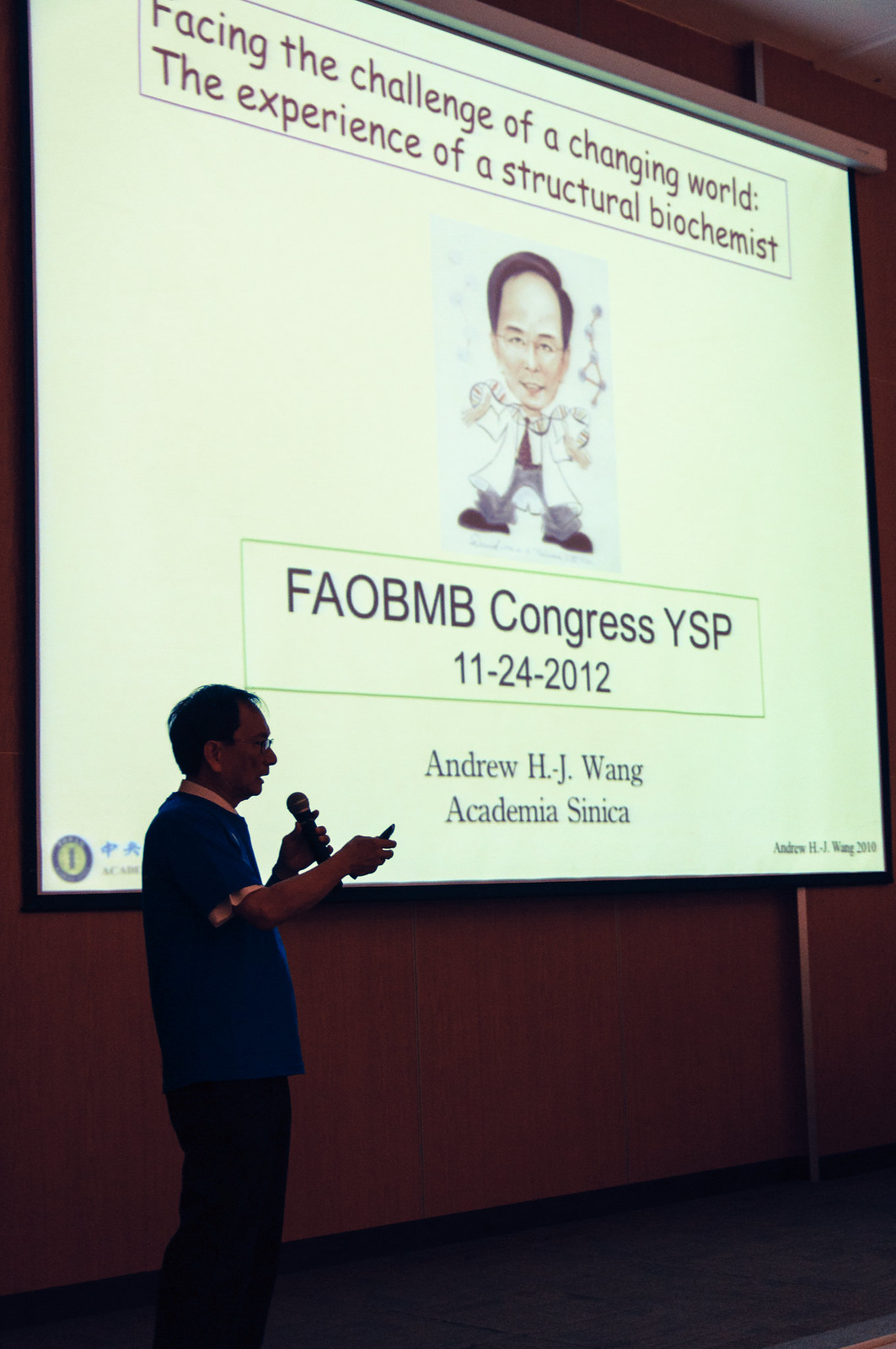In the image, we see an older man standing at the front of a lecture hall, delivering a presentation. He is depicted holding a microphone in his left hand and a piece of paper or possibly a remote control in his right hand. The man is dressed in a blue shirt with white trim around the collar and sleeves, over a white t-shirt, and paired with dark pants. He stands before a large projector screen, which casts a shadowy outline of him onto the wall. The room is dimly lit, with dark gray or blue flooring and maroon-colored walls. The projector screen prominently displays the text "Facing the Challenge of a Changing World: The Experience of a Structural Biochemist" at the top, accompanied by a cartoon-like illustration of a man in a lab coat surrounded by molecules and beakers. Beneath the illustration, the text reads, "FAOBMB Congress, YSP 11-24-2012, Andrew H. J. Wang, Academia Sinica." The colors in the image include shades of blue, white, tan, gray, and black, with the presentation screen being a central focal point of the scene.